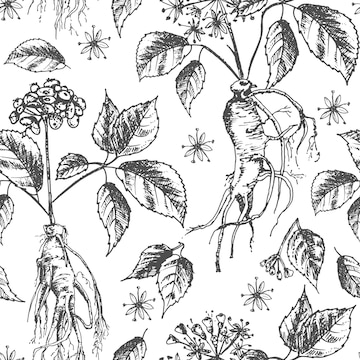The image depicts a detailed digital, monochrome line drawing primarily featuring carrot plants. The drawing includes well-defined roots at the bottom and leafy tops, with several individual carrots shown in various orientations. Scattered around the main subjects are floating leaves and budding flowers, all intricately rendered. The artwork, composed entirely of black lines set against a white background, is designed for potential use in various decorative applications such as fabric or wrapping paper, inviting the possibility of adding personal color. This repetitive yet elegant pattern showcases a range of botanical elements, blending root vegetables and floral motifs seamlessly across the canvas.